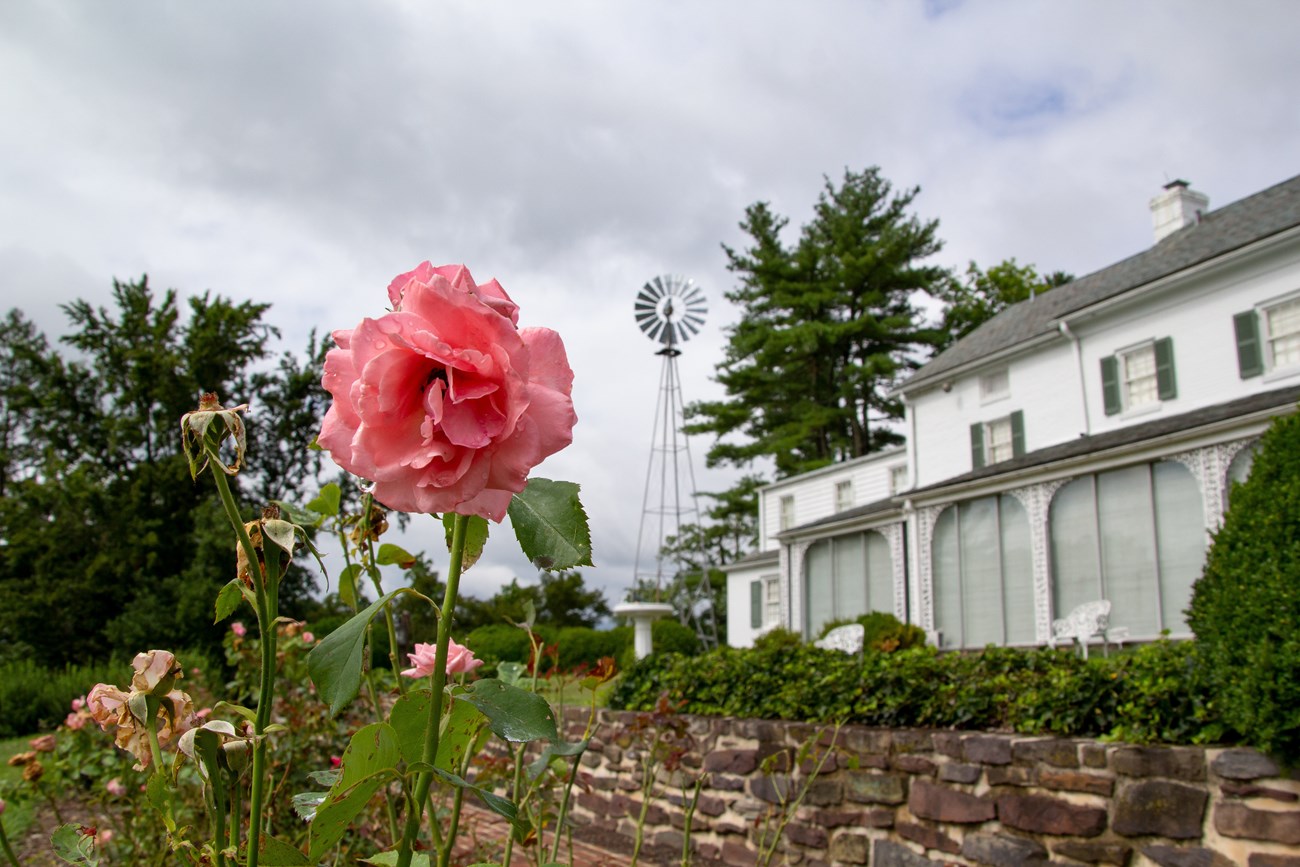In this image, the main focus is a large, vibrant pink rose prominently positioned slightly to the left. Surrounding it are various rose bushes, with most of the flowers wilted except for another live rose in the distance. The scene is set in a lush, green grassy area with multiple trees and shrubs. To the right stands a striking white farmhouse characterized by arched windows with blue panels on the second story and a chimney on the roof. This colonial-style house is accompanied by a long brick wall topped with shrubs, and a white birdbath is visible in the vicinity. Flanking the scenery, a large weathervane-type structure, reminiscent of a windmill, punctuates the cloudy sky, adding a rustic charm. The overall ambiance is tranquil yet somber, with the overcast sky casting a diffused light over the picturesque yet slightly melancholic landscape.